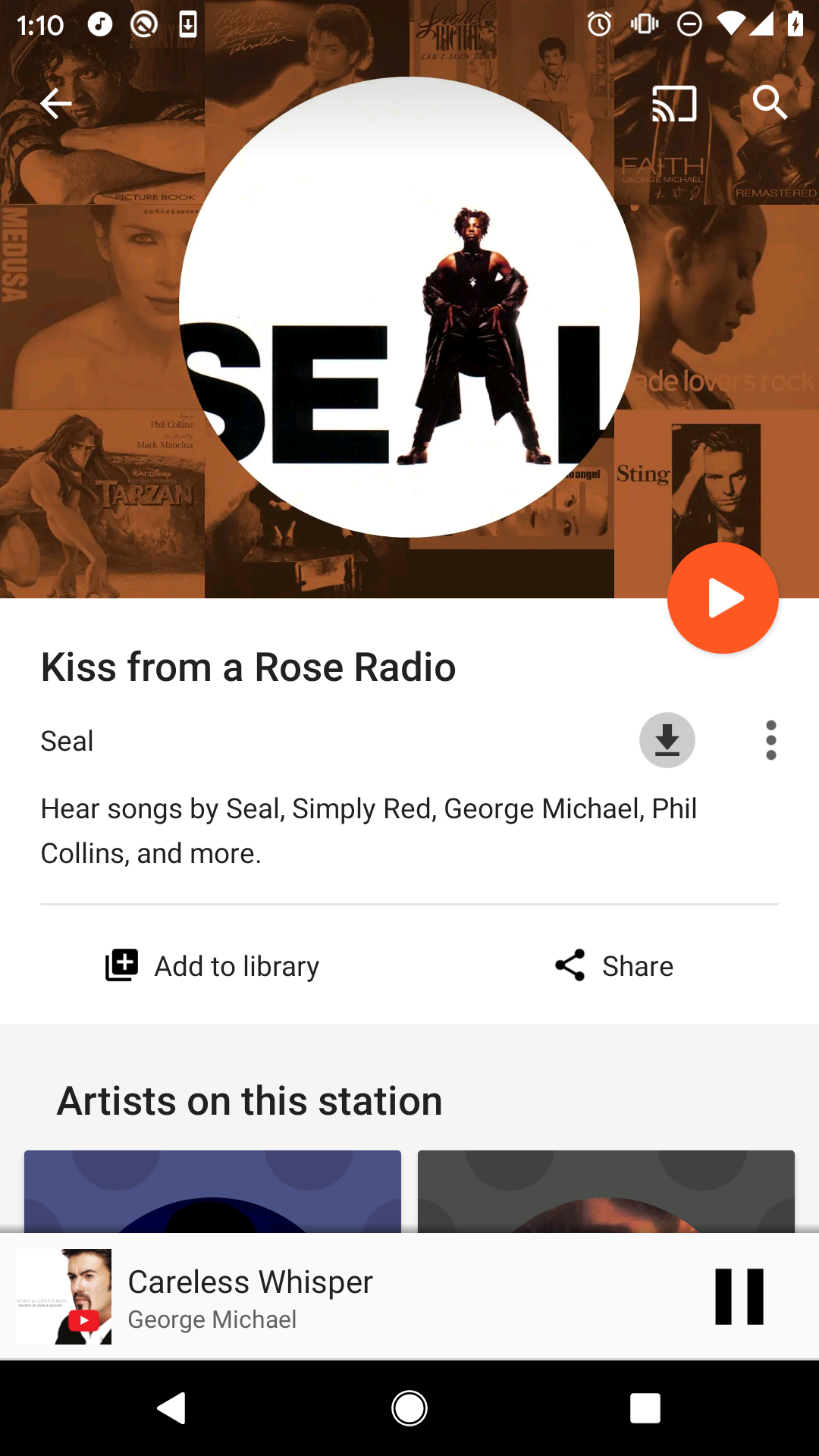This screenshot captures an interface from either an online radio app or a music player app. The screen displays the time as 1:10, along with various icons including a music note within a circle, a download button, an alarm, a vibration icon in a circle, full Wi-Fi and signal strength indicators, a full battery icon, a screen share button for casting to a TV, and a magnifying glass for search. There's also a back arrow positioned on the left side of the interface.

The background features a montage of album covers in sepia tones of orange, black, and gray. Prominently displayed in the center is a white circle with the name "Seal" written inside. The "A" in "Seal" is creatively formed by Seal standing with his legs apart, dressed in a long jacket, baggy pants, and a sleeveless tank top, exuding a bold stance.

If it's not Seal himself, it’s an artist designed to look like him. Adjacent to his name is the title "A Kiss from a Rose." There's a prompt indicating that you can download the song, listen to more tracks by Seal, Simply Red, George Michael, Phil Collins, and others. The options to add the song to your library or share it are also present. An orange circle with a white play button sits just below this header image.

Below, there's a section listing artists on this station, though the images on the left and right are indistinguishable. Beneath, an image of George Michael is visible with the title "Careless Whisper" and a pause button next to it, indicating the song is currently playing. Finally, at the bottom of the screen is a black navigation menu.